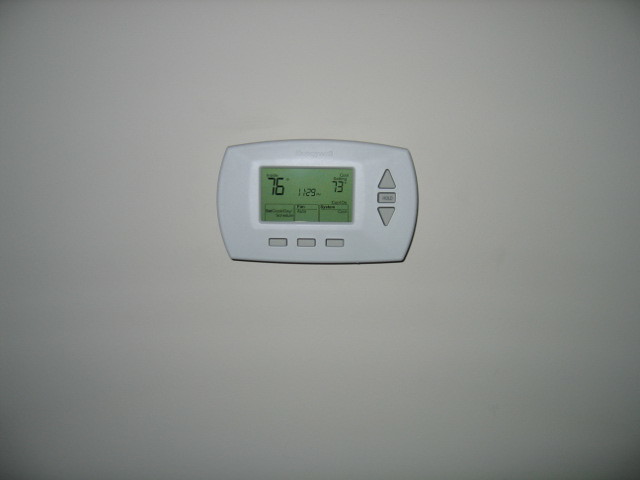The image depicts a plain white wall, serving as the background for an air conditioning and heating control unit. The unit is white and features a digital display. The display unit is approximately 14 centimeters wide and 24 centimeters high. On the right side of the control, there are three gray buttons: an upward-pointing triangle, a "HOLD" button, and a downward-pointing triangle beneath it.

Directly below the rectangular display are three unmarked gray rectangle buttons. The display shows the indoor temperature, which is 76 degrees Fahrenheit, and the set temperature at which the system will activate. The current time displayed is 11:29 p.m. The fan is set to auto, and the unit is configured to cool. The digital display has digitized numbers with a greenish-grayish tint. Other items on the display are not clearly readable.